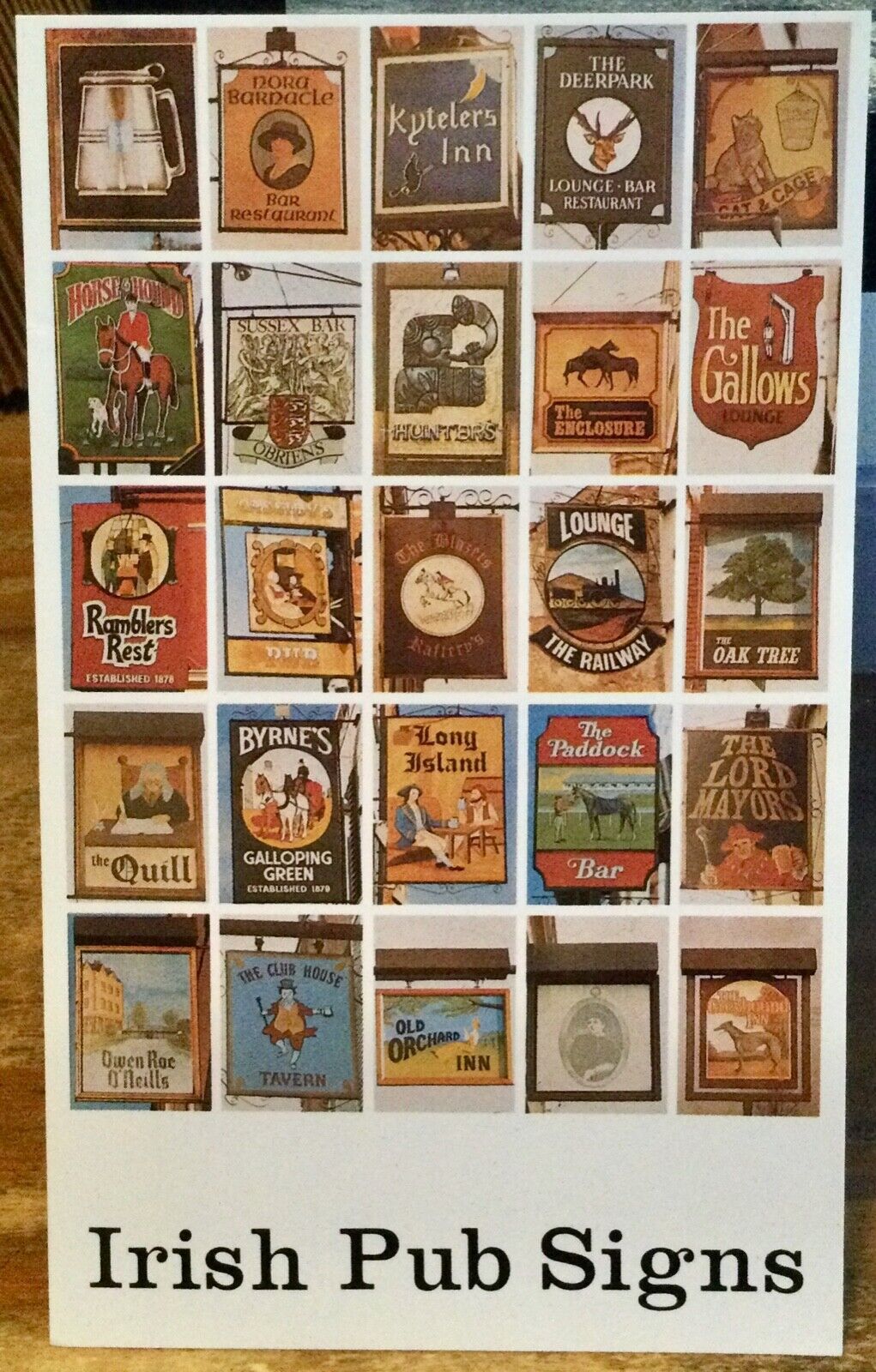This image showcases a collage of 25 distinct Irish pub signs, arranged in a 5 by 5 grid against a white background. At the bottom, in black text, it reads "Irish Pub Signs." Each sign occupies an individual block and features unique and colorful artwork representative of the pub's name and character. Notable examples include the "Nora Barnacle Bar and Restaurant" with a lady wearing a hat, "Kytellers Inn" with a raven on a branch, "The Deer Park Lounge Bar and Restaurant" featuring a deer head with antlers, and the "Cat and Cage" with a cat looking up at a cage. Additional signs include "Horse and Hound" depicting a rider and a dog, "The Gallows" with an image of a gallows, "Rambler's Rest," "The Oak Tree," "Lounge the Railway," "The Paddock Bar," and "The Lord Mayor’s," among others. The designs range from intricate illustrations to simple yet evocative imagery, capturing the rich heritage and charm of Irish pubs.